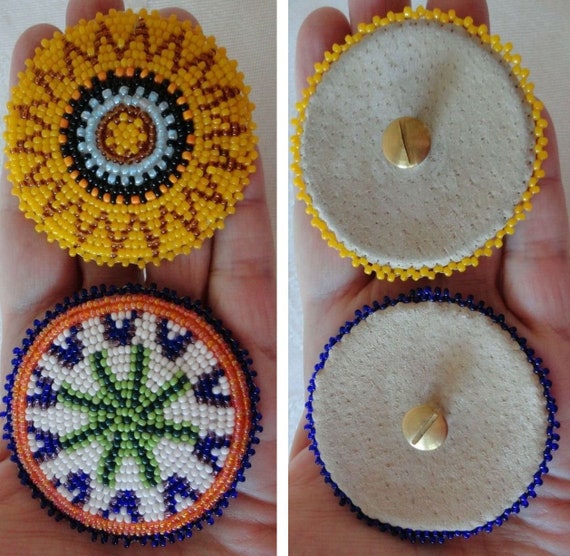This color photograph features a close-up of someone's hand holding two intricate, circular beadwork designs, reminiscent of Native American artistry, displayed against a neutral background. On the left side, the top design resembles a radiant sun, where the outer edge is predominantly yellow with a striking red zigzag pattern, reminiscent of rays of the sun. Moving inward, the design transitions to orange, black, and white, culminating in a yellow center. The bottom left design features a border of blue and orange, framed around a central motif that starts with blue and transitions to white. Within these borders, two rows of red beads encase a pattern with blue elements and a flower-like design of light and dark green hues at its nucleus. On the right side, the photo shows the back, revealing a white, textured material possibly made from suede leather, with visible metal screw tops suggesting these designs can be attached to items. The detailed craftsmanship and the handheld scale of the items highlight their delicate and compact nature.